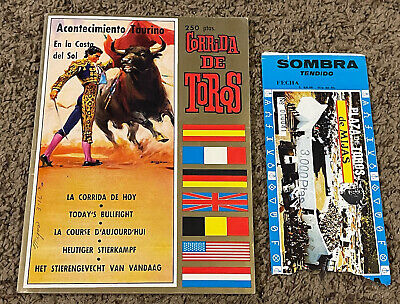The photograph depicts a brown bullfighting brochure and a partially ripped ticket stub, both lying on a brown carpet floor. On the left, the brochure features the title "Corrida de Toros" in red font at the top right corner. Below this title, seven international flags are displayed, including those of Spain, France, Mexico, the United Kingdom, Germany, the United States, and an unidentified one, suggesting an international event. The central image on the brochure shows a dramatic scene of a matador and a charging bull. The matador, dressed in a traditional black and gold suit with pink socks and black shoes, holds a red cape in his left hand and a sword in his right, with sand kicking up around them in the arena. The background of the brochure has a goldish-tan hue. To the right of the brochure is a blue ticket stub with black lettering, indicating seat details and potentially the cost, partially torn, implying prior use. The ticket has "Sombra Tiendillo" written on it, among other Spanish phrases, situating it firmly in the context of a bullfight event.